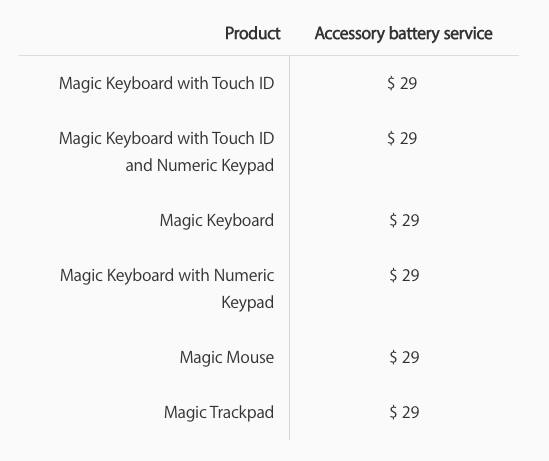The image showcases a product and accessory battery service pricing guide against a light gray, nearly white background. The guide is organized into two vertically-aligned columns, with each column clearly labelled at the top. The left column is titled "Product," and the right column is titled "Accessory Battery Services Center."

The product details in the left column are left-justified, creating a neat and orderly appearance. A thin gray horizontal line at the top separates the titles from the contents below, while another thin gray vertical line divides the two columns.

Listed under the "Product" column are various Apple accessories, each followed by their respective service price of $29. The items are as follows:
1. Magic Keyboard with Touch ID - $29
2. Magic Keyboard with Touch ID and Numeric Keypad - $29
3. Magic Keyboard - $29
4. Magic Keyboard with Numeric Keypad - $29
5. Magic Mouse - $29
6. Magic Trackpad - $29

The structured layout and clear delineation of information make it easy for customers to identify both the product and the associated accessory battery service price.